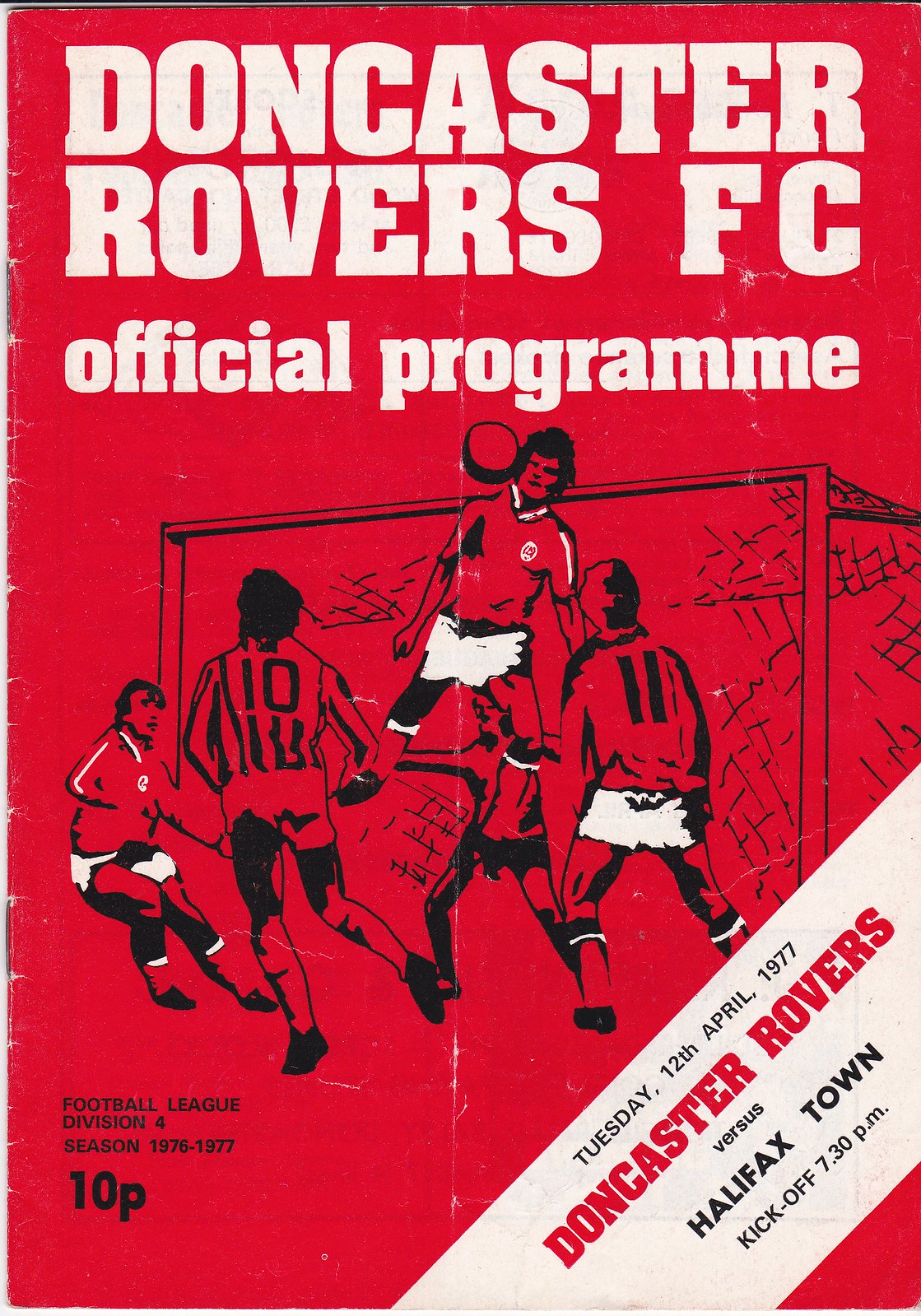This is an image of the front cover of a football (soccer) program for a match between Doncaster Rovers and Halifax Town. The cover features a bold red background with large white letters at the top that read "Doncaster Rovers FC Official Program." Below this text, there is a detailed black and white illustration depicting an intense moment in a soccer match. The graphic shows a goalkeeper leaping into the air to block an incoming ball, while four other players are engaged in the play. Two of the players, seen from the back, are wearing jerseys numbered 10 and 11. The players' shorts are white, providing a stark contrast against the red background. At the bottom left corner, there is text that reads "Football League Division 4, Season 1976-1977, 10-P." In the bottom right corner, a white diagonal banner states, "Tuesday, 12 April 1977, Doncaster Rovers vs. Halifax Town, Kickoff 7.30 p.m." This program is a visual indicator of an upcoming football match from the 1976-1977 season.